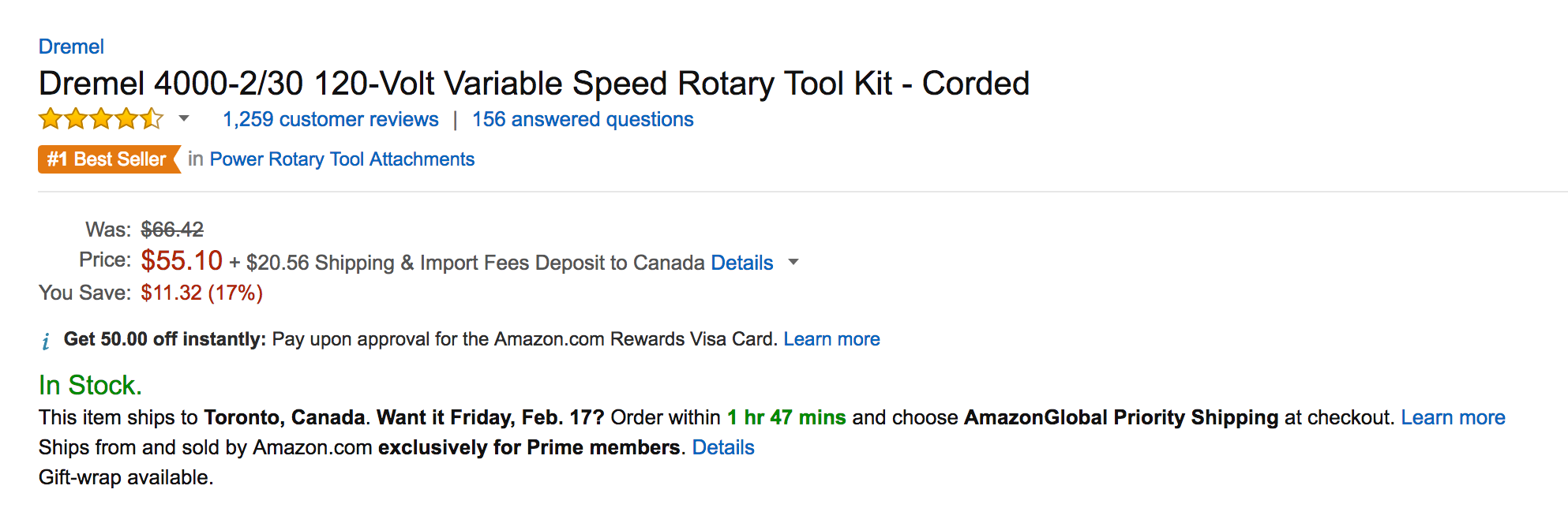**Product Listing Screenshot: Dremel 4000-2/30 120-Volt Variable Speed Rotary Tool Kit - Corded**

This screenshot captures a detailed listing for the Dremel 4000-2/30 120-Volt Variable Speed Rotary Tool Kit on Amazon. At the top, the product brand "Dremel" is displayed in blue letters, followed by the product name in bold black font. 

**Product Details:**
- **Rating:** 4.5 out of 5 stars, based on 1,259 customer reviews.
- **Customer Interactions:** 156 answered questions, both of which are hyperlinked for further details.
- **Category:** Number 1 bestseller in Power Rotary Tool Attachments, with clickable links for customer reviews, answered questions, and the category itself.

**Pricing Information:**
- **Original Price:** $66.42
- **Current Price:** $55.10
- **Additional Costs:** $20.56 for shipping and import fees deposit to Canada
- **Savings:** $11.32 (17% off the original price)
- **Special Offer:** Get $50 off instantly upon approval for the Amazon.com Rewards Visa Card (clickable link for more details).

**Availability:**
- **Stock Status:** In stock (indicated by green text).
- **Shipping Information:** Ships to Toronto, Canada. 
- **Expedited Shipping Option:** Available with Amazon Global Priority Shipping; order within 1 hour and 47 minutes to receive by Friday, February 17th (in green text, with a clickable link for more details).
- **Seller Information:** Ships from and sold by Amazon.com, exclusively for Prime members (link for details).
- **Gift Wrap:** Available option.

This organized and detailed caption provides a comprehensive overview of the product listing, including price details, customer interactions, and shipping information.